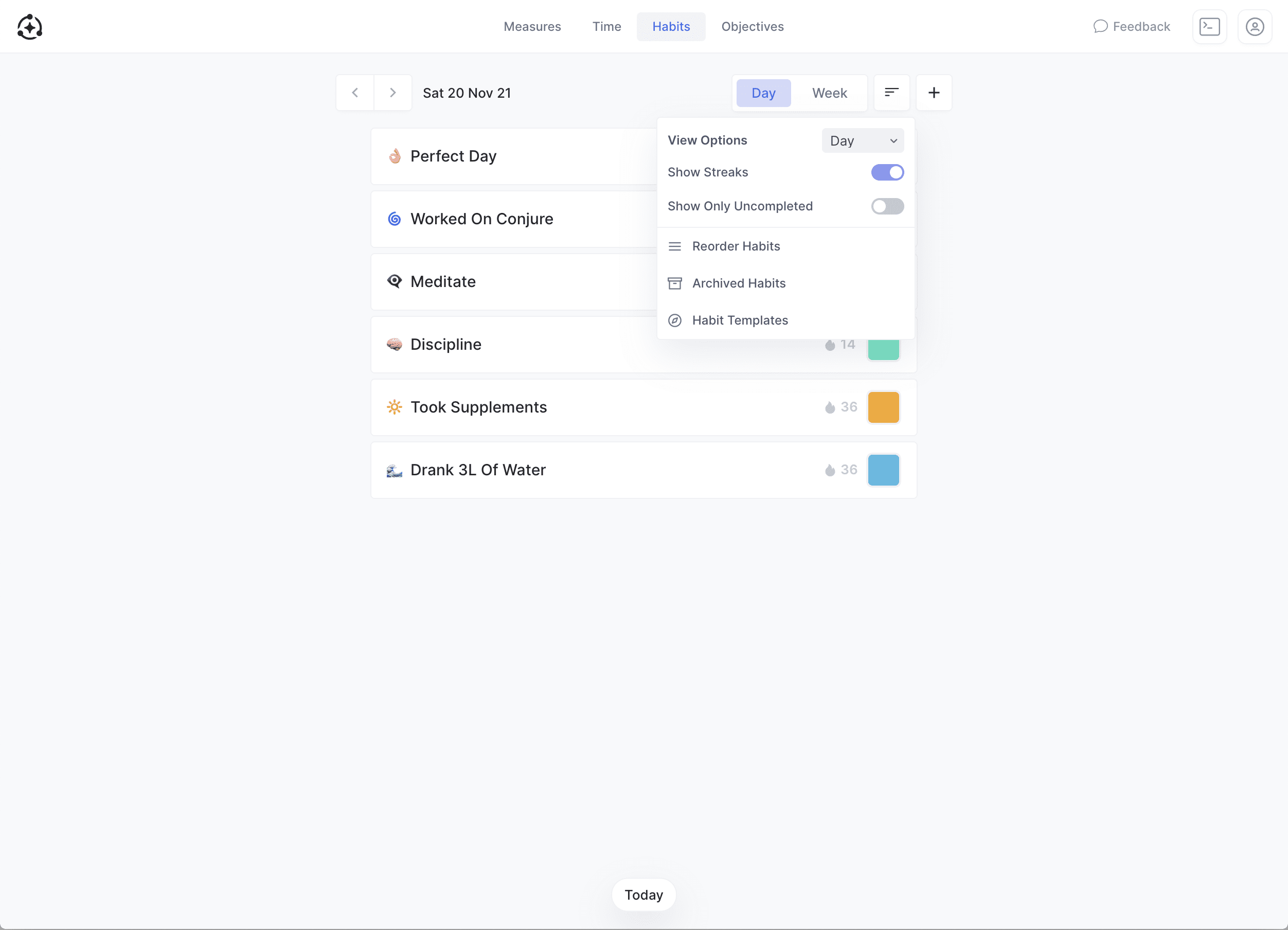Certainly! Here’s a cleaned up and detailed caption for the image you described:

---

On a grey background, there is a detailed interface for tracking measures, time, habits, objectives, and feedback, predominantly highlighted in blue. 

- At the top, a highlighted blue square contains the text "Saturday, SAT 20 NOV 21," indicating the specific date.
- Below the date, navigation options labeled "Day" and "Week" are displayed, with "Day" highlighted in blue.
- A square to the left features a profile icon with left and right arrows for navigation.
- Adjacent to this, another square, framed by a blue border, showcases three lines of increasing length from bottom to top, representing progress.
- To the right, a square with a plus sign is visible.

Further down, segmented sections reveal different habit progressions:
- The section titled "Perfect Day" lists activities such as "Worked on conjure," "Meditate," and "Discipline." While most sections are obscured by a white overlay, the "Discipline" section shows the number 14.
- The "Took Supplements" habit is marked with a thumbs-up icon and the number 36.
- Habit icons include a yellow square for "Discipline" and a green square for "Drink 3L of Water," both marked with a thumbs-up icon and the number 36.
- There's another notation with a blue square.

At the bottom of the interface, a white oval button labeled "Today" stands out.

Lastly, a white box marked "View Options" includes toggles for additional settings, such as "Show Streets" (turned on) and "Show Only Uncompleted" (turned off).

---

This caption provides a clearer, more structured description of the image’s content.